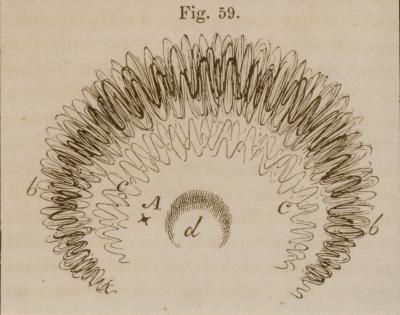Figure 59 is a detailed black-and-white illustration, likely extracted from a book or academic paper. The drawing resembles a dandelion or a spirograph pattern, characterized by a series of concentric half-circles created by dense, squiggly lines. The illustration is meticulously labeled: the outermost wave, marked as 'B,' consists of more prominent and denser lines with significant highs and lows, giving it a star-like appearance. Just inside of 'B,' the waves labeled 'C' are softer in intensity. At the very center is the letter 'D,' representing the innermost layer, which features much finer, scratch-like lines. Additionally, the letter 'A,' which is an uppercase, is placed near the center next to 'D.' The background is white, and the print is entirely in black, ensuring high contrast and clarity. The illustration is precise and deliberate in its pattern, suggesting it could be an etching done with a spirograph or a diagram of a vocal apparatus, emphasizing the illustration's structured nature rather than randomness.